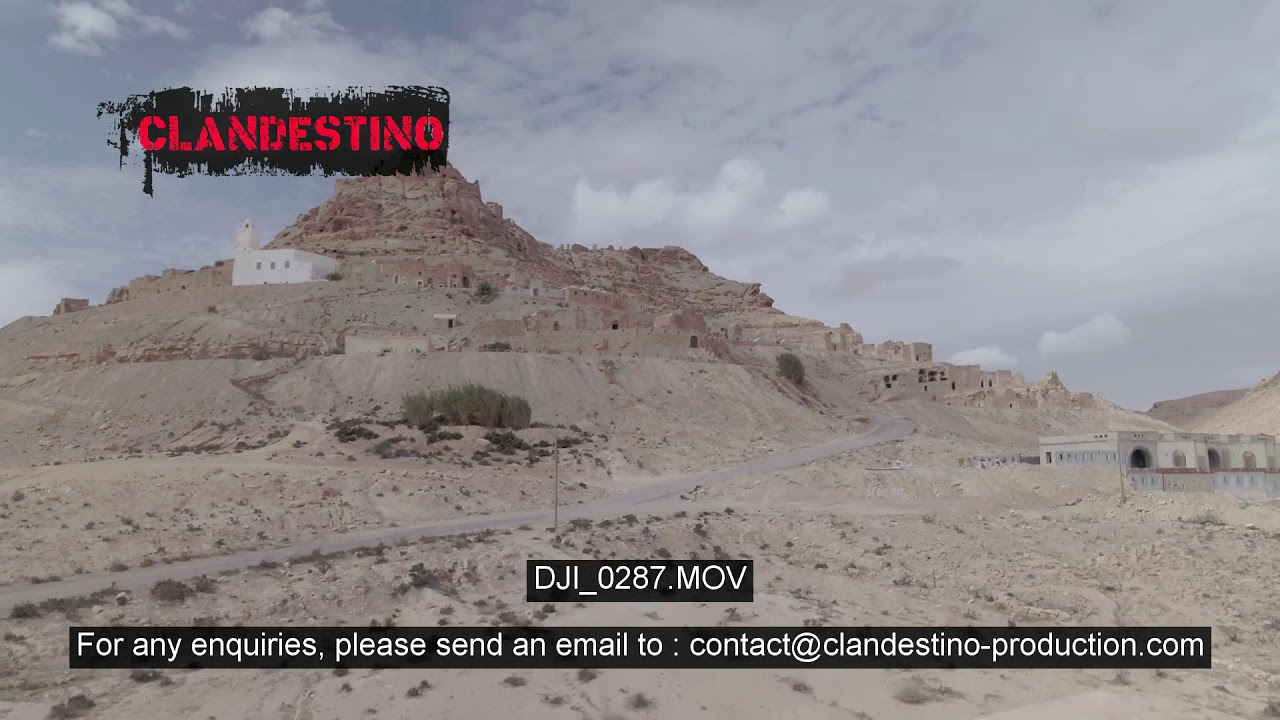The image depicts a desolate desert landscape dominated by dry sand and a tall, rocky hill. At the summit of the hill, a distinct white building with three windows stands out. A pathway leads up to the rocky mountain, where more stucco buildings are nestled against its lower slopes. The cliffs in the background, appearing as gray stone tiers, house several shoebox-like structures with small openings, suggesting the remnants of ancient ruins. Sparse green bushes can be seen at the base of the ruins. In the upper left corner, red text reads "Clandestino," set against a black, paint-like backdrop. The bottom of the image features white text that reads "DJI 0287.MOV" alongside a note inviting inquiries via email to contact@clandenstinoproduction.com.